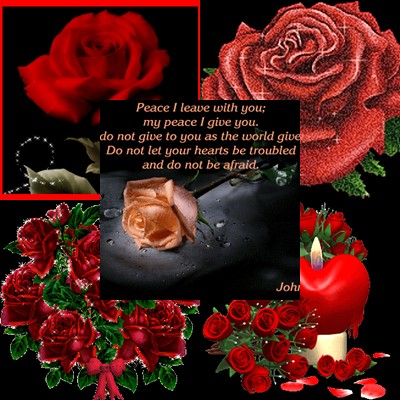The image is a meticulously crafted composite of five different photographs, arranged in a four-quadrant layout with an additional central overlay. Each quadrant portrays a unique depiction of roses against a black background:

1. The upper left quadrant features a strikingly realistic red rose with rich, ruby petals and vivid green leaves, bordered in red.
2. The upper right quadrant displays a sparkling, cartoonish red rose, set against a black backdrop with hints of green leaves.
3. The lower left quadrant showcases a wreath of green leaves intertwined with multiple cranberry-colored roses, adorned with a matching cranberry bow.
4. The lower right quadrant shows a bouquet of roses next to scattered petals and a partially blacked-out lit candle, suggesting a heartfelt scene.

At the center of this quadrant arrangement lies a black overlay square, prominently featuring an orange rose on a grayish-black background. Inscribed in peach-colored text is a poignant biblical passage: "Peace I leave with you, my peace I give you. Do not give to you as the world gives. Do not let your hearts be troubled and do not be afraid." The text, attributed to John, expresses a comforting message of peace and reassurance.